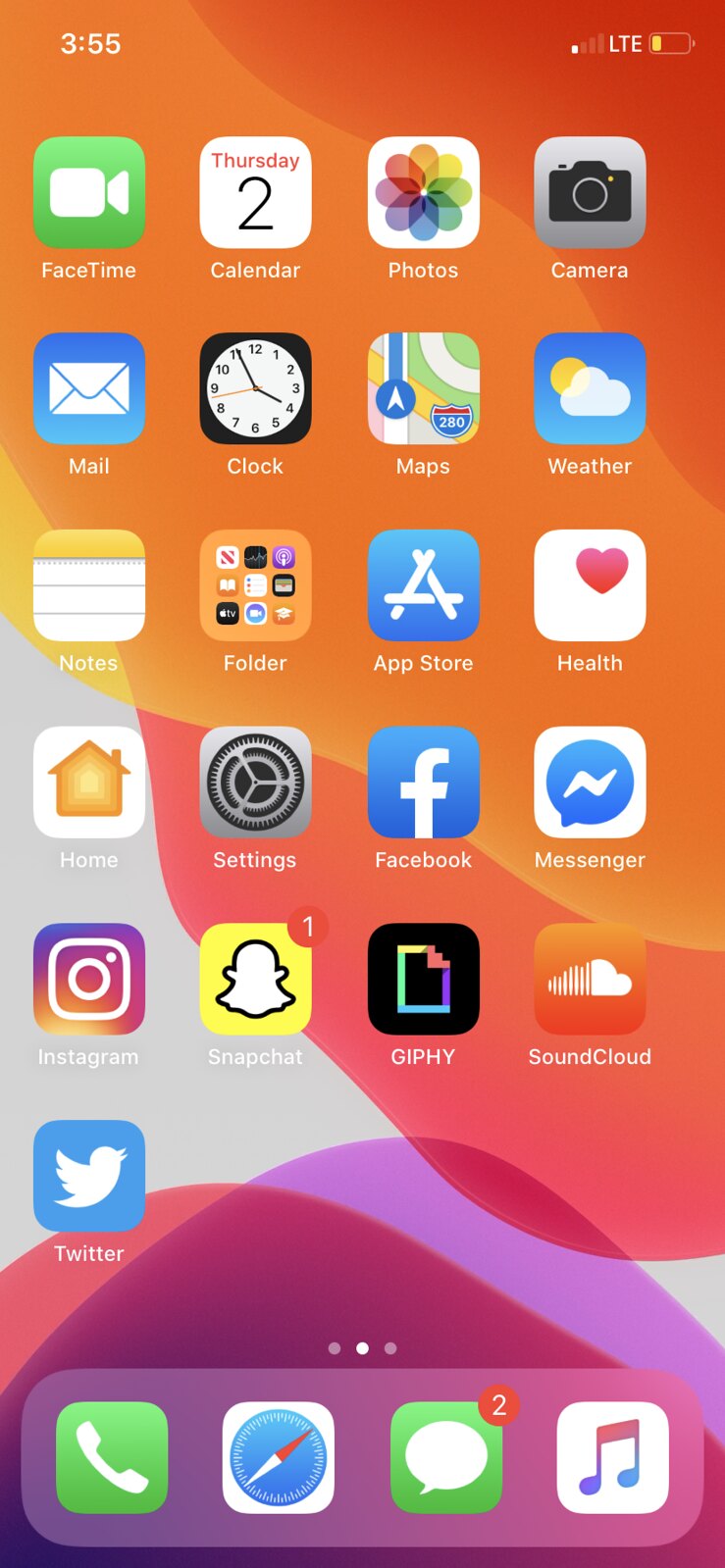The image shows the home screen of a smartphone. In the top right corner, the LTE signal icon and a nearly depleted battery indicator are visible, with the time displayed as 3:55. Prominently featured app icons include:

- **FaceTime**: A green icon with a white video camera symbol.
- **Calendar**: A white icon displaying "Thursday 2nd" in black text.
- **Photos**: A colorful icon resembling a flower with red, blue, yellow, and green petals.
- **Camera**: A black camera inside a silver square.
- **Mail**: A white envelope on a blue background.
- **Clock**: A black icon with a white clock face.
- **Maps**: A multicolored map icon.
- **Weather**: A blue square with a white cloud and yellow sun.
- **Notes**: A yellow notepad icon.
- **App Store**: A white "A" on a blue background.
- **Health**: A white icon with a red heart.
- **Home**: An orange icon resembling a house.
- **Settings**: A gray gear icon.
- **Social Media and Other Apps**: Icons for Facebook, Messages, Instagram, Giphy, SoundCloud, and Twitter are also visible.

Additionally, the Messages app icon indicates there are two unread messages.